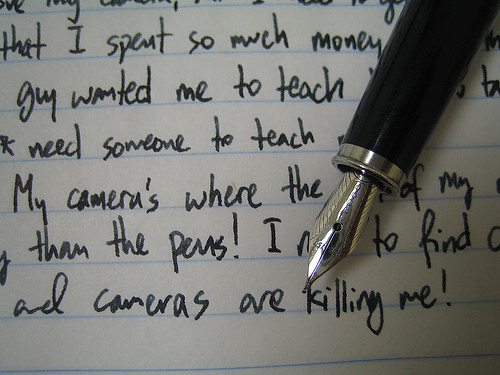The image features a square, photograph of a white piece of college-ruled notebook paper with light blue horizontal lines. Handwritten text on the paper appears to be part of a narrative, with legible phrases such as "I spent so much money," "guy wanted me to teach," and "cameras are killing me," though some parts of the text are illegible due to the positioning of an old-fashioned, black fountain pen with a silver, etched tip. The pen is placed diagonally from the top right-hand corner towards the bottom left. The image is somewhat dark, especially in the lower right-hand corner, suggesting poor lighting in that area. The focus of the photograph seems to highlight both the handwritten note and the intricate design of the fountain pen.